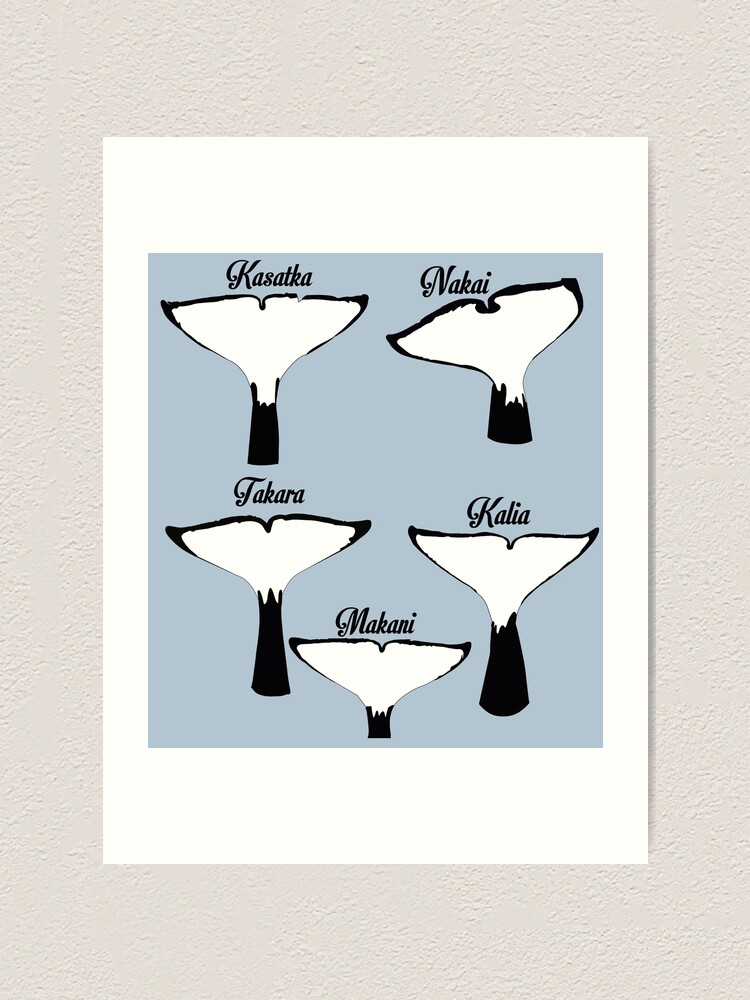This artwork is a poster of five illustrated whale tails, prominently featuring a blue background with black and white tails. Each tail is labeled above with names including Kasatka, Nakai, Takara, Makani, and Kalia. The poster, enclosed in a thick white border on the top and bottom and a slimmer white border on the sides, is hung on a white, popcorn-textured wall. The tails, likely of orca whales, are each slightly different, showcasing a customization in their illustrations. The names, written in black script, are carefully placed above each respective tail, suggesting identification of each individual whale.